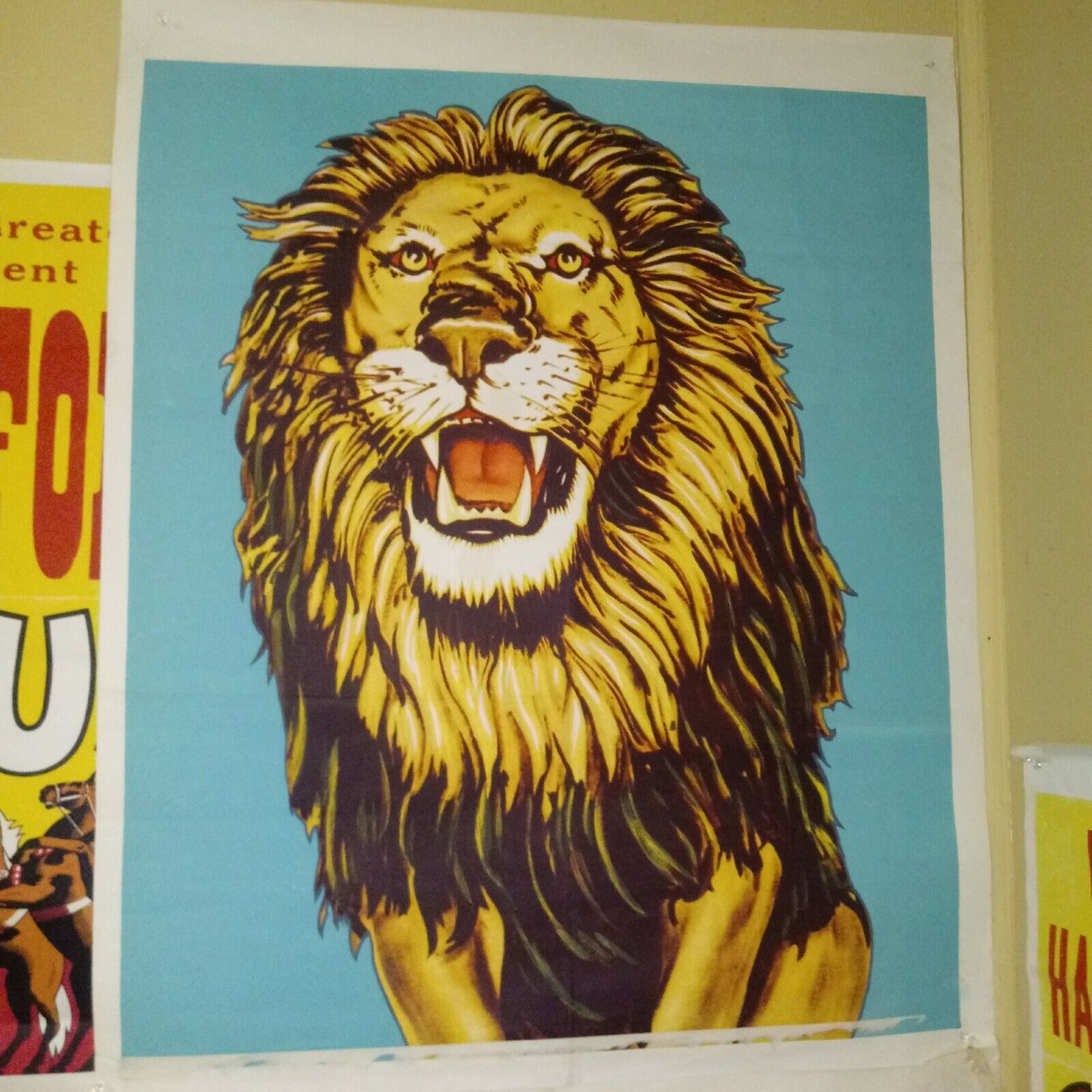The image shows a vertically-oriented, slightly faded poster hanging on a yellow, plastered wall. The central figure on the poster is an artistically rendered male lion, depicted in shades of yellow with a fully flowy mane, against a blue background with white borders. The lion is sitting on its haunches, with its mouth open wide in a roar, showcasing four long, prominent fangs. The poster seems to capture a top-down view of the lion’s face and flowing mane, with some of its lower feet visible. Surrounding the lion, parts of another poster are visible, with one on the left suggesting a circus theme, featuring trained horses rearing up on their hind legs.